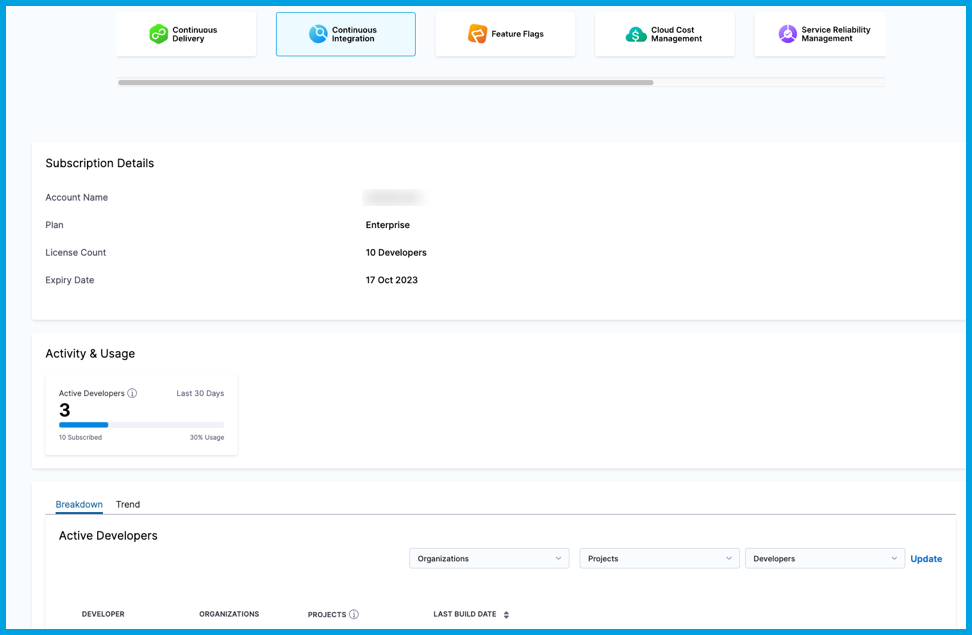**Detailed Caption**: 

The image is a screenshot from an unspecified digital platform, outlined by a blue border and set against a white background. At the top, the section titled "Continuous Delivery, Continuous Integration" is highlighted, indicating it has been selected. Other visible options include "Feature Flags," "Cloud Cost Management," and "Service Reliability Management."

A gray horizontal line separates this section from the "Subscription Details" below. The account name in this section is blurred out for privacy. The subscription is labeled as an "Enterprise" plan with a license count for 10 developers. The subscription is set to expire on 17 October 2023.

Below, under "Activity and Usage," it indicates that there are 3 active developers out of 10 subscribed in the last 30 days, reflecting a 30% usage rate. The "Breakdown" tab is also selected here, and it leads to further details such as "Trend," "Active Developers," "Organizations," "Projects," and "Developers" which are options for more specific data analysis.

Towards the bottom of the image, additional categories are listed: "Developer," "Organizations," "Projects," and "Last Build Date."

The image contains no photographical elements, people, animals, birds, plants, flowers, trees, buildings, automobiles, or airplanes, indicating a purely graphic and text-based content with a focus on subscription and usage analytics.